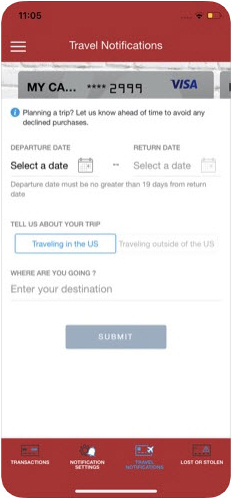The image captures a screenshot of a travel app displayed on an Apple iPhone, characterized by maroon red UI bars at the top and bottom. The status bar at the top displays the time "11:05" in black text, along with a Wi-Fi icon and a battery indicator at approximately 50%.

The bottom of the screen features a navigation bar with four buttons, each accompanied by icons and white text: "Transactions," "Notification Settings," "Travel Notifications" (highlighted in blue), and "Lost or Stolen." Below this, the white Apple home line is visible.

At the very top of the app interface, a hamburger menu icon is positioned beside a white title that reads "Travel Notifications." The central portion of the screen contains a form for setting travel notifications. The top of the form displays an image of a Visa card, labeled "myca****2999," with the Visa logo appearing prominently. The card image is partially obscured by the rest of the content below.

The form includes fields and buttons for entering travel details:
- "Departure Date: Select a date"
- "Return Date: Select a date"
- A button labeled "Traveling in the US"
- A field "Where are you going?"
- A field "To your destination"
- A "Submit" button

The interface is designed to collect travel information, ensuring that the user's credit card is aware of their travel plans to avoid any interruptions in service.